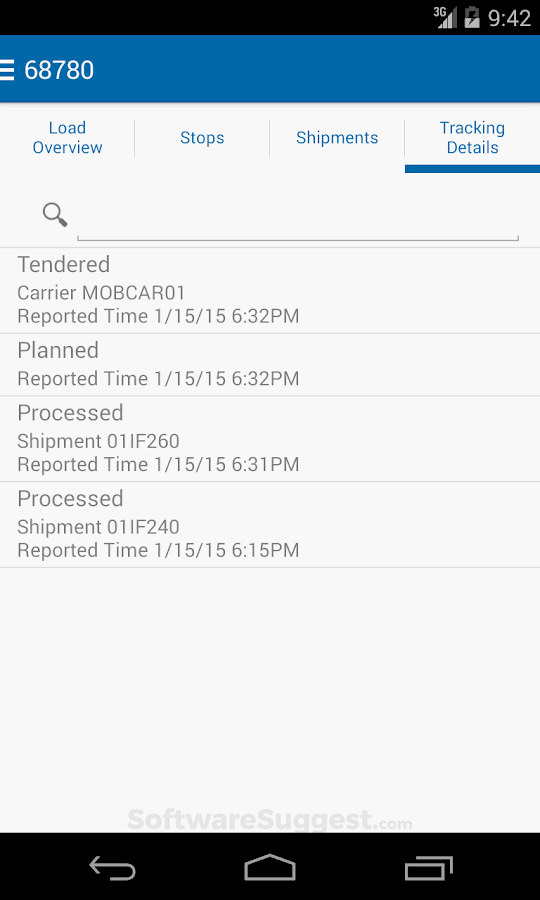Here is a cleaned-up and detailed caption based on the provided description:

---

The image is a screenshot of an Android phone, evidenced by the distinct style of the icons at both the top and bottom of the screen. The upper portion features a black horizontal bar, which is mirrored by another black horizontal bar at the lower end of the display. 

In the middle to the top of the screenshot, a blue bar is visible with white text and symbols. On the left side of this bar, there are three horizontal lines stacked on top of each other, indicating a menu button. Adjacent to this, the number "68780" appears, which seems to be a zip code. Beneath this section, several menu options are listed: "Load Overview," "Stop," "Shipments," and "Tracking Details."

Directly below these menu options, there is a magnifying glass icon, typically used for searching. Next to it is a box icon. Further down, the screen displays four rows, each with grouped information. The rows are labeled as follows:

- "Tenured Carrier"
- "Reference, Reported Time, Date, Time, Planned"
- "Report Time, Date, Time, Processed Shipment"
- "Identifier, Report Time, Date, Time, Processed Shipped"

At the very bottom of the screen, the text "software suggest.com" is displayed.

---

This polished caption provides a detailed and organized description of the particular screenshot from the Android phone.